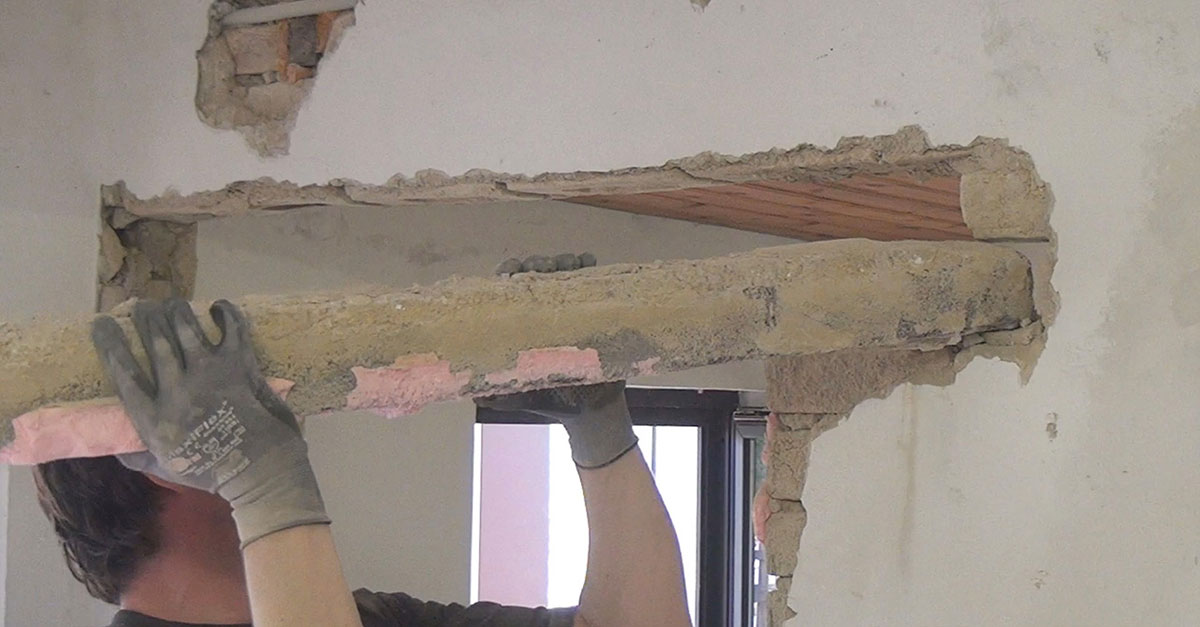The image depicts an individual inside a home engaged in renovation work. A Caucasian man with short brown hair, wearing a black shirt and black gloves, is in the process of demolishing part of a white plastered concrete wall. He is holding a long piece of concrete, suggesting he is either removing or tearing down sections of the wall. In the top left corner of the image, damage to the wall reveals underlying bricks and concrete fragments. This indicates the creation of an archway or a large opening for further construction. In the background, there is a window with daylight filtering through, highlighting that the activity is taking place during the daytime.